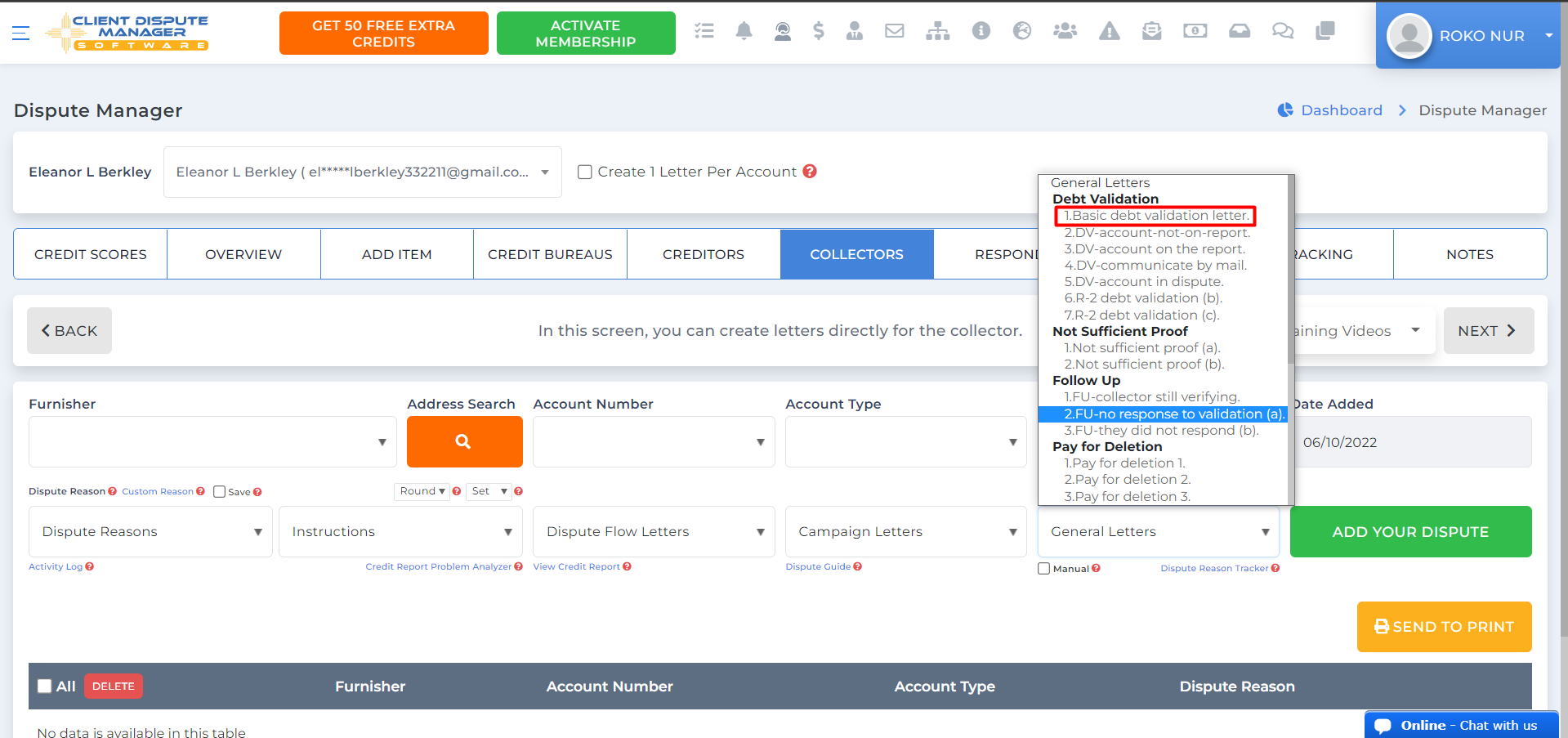This image captures a webpage for "Client Dispute Manager Software," prominently displayed in the top left corner. Adjacent to the title, an orange rectangle with white text offers "Get 50 Free Extra Credits," and beside it, a green rectangle urges users to "Activate Membership." In the top right corner sits a blue rectangle, featuring a circular avatar space next to the name "ROKO NUR" in capital letters. 

On the left side, the text "Dispute Manager" appears in black, with "Eleanor L Berkeley" listed underneath, accompanied by a dropdown box displaying her name and email address. Below this, a prompt reads "Create One Letter Per Account."

Further down, a series of tabs includes "Credit Scores," "Overview," "Add Item," "Credit Bureaus," "Creditors," "Collectors" (highlighted in blue), "Response," "Tracking," and "Notes." Additional dropdowns include "Furnisher," "Address Search," "Account Number," "Account Type," "Dispute Reasons," "Instructions," "Dispute Flow Letters," "Campaign Letters," and "General Letters."

At the bottom of the page, two prominent buttons stand out: a green rectangle labeled "Add Your Dispute" and a yellow rectangle labeled "Send to Print."